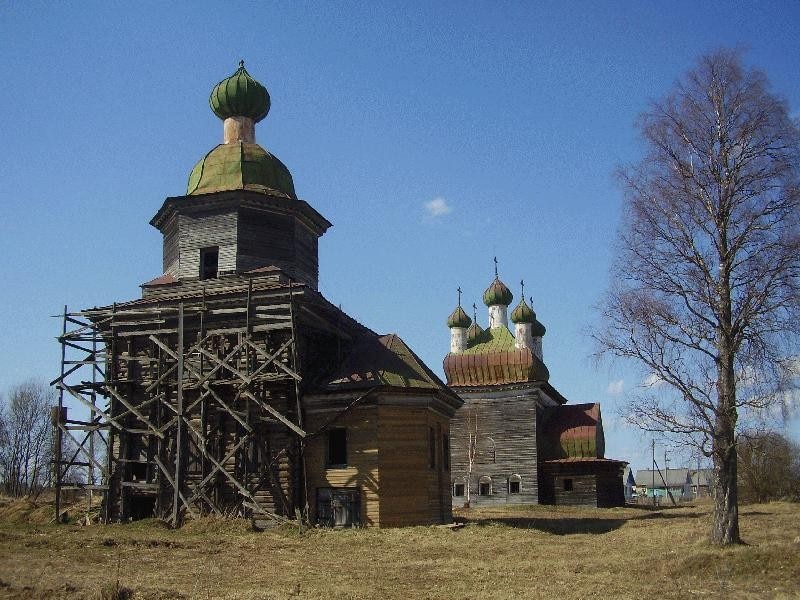The photograph captures a serene autumn scene with a vivid blue sky dotted by a few thin white clouds. Dominating the foreground are two old wooden buildings, showcasing distinct Russian architectural elements with their green domes and bulbous spires topped by crosses. The closest building, partially encased in wooden scaffolding and suggesting ongoing renovations, features a main spire and a doorway, constructed from dark wood that contrasts with newer wood on its walls. The second building, positioned slightly further and to the right, is larger and adorned with five ornate spires. Below this charming skyline, the grass lawn appears beige, indicating late fall, and is surrounded by an array of leafless trees. On the far right, one tall, thin, gray tree stands prominently, while in the background on both sides, more trees and low, rectangular buildings with gray roofs can be seen, all basking under the daylight sun.